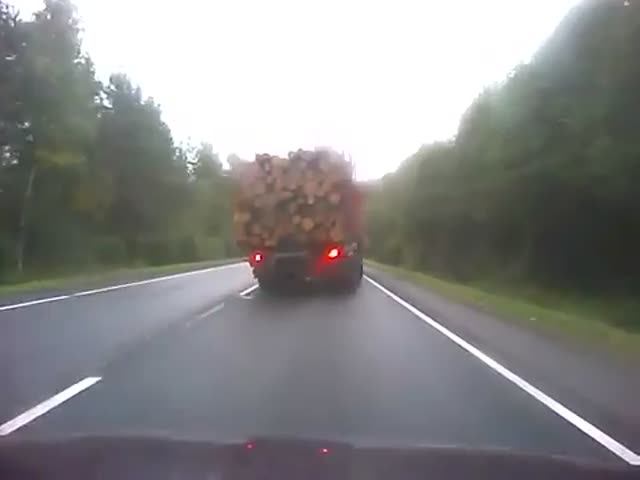The blurry image is taken from the front seat of a vehicle on a two-lane highway, prominently featuring the back of a large truck heavily loaded with neatly stacked brown tree logs. Only the very tip of the vehicle’s hood is visible at the bottom of the scene. The highway has solid white lines on either side and a dashed white line in the center. Surrounding the road are green trees, indicative of a spring or summer setting, and grassy embankments slope down from the road. All the truck's brake lights are illuminated in red, suggesting it might be slowing down or stopping. The sky appears white, possibly due to cloud cover or the image's blurriness, making precise details hard to discern.